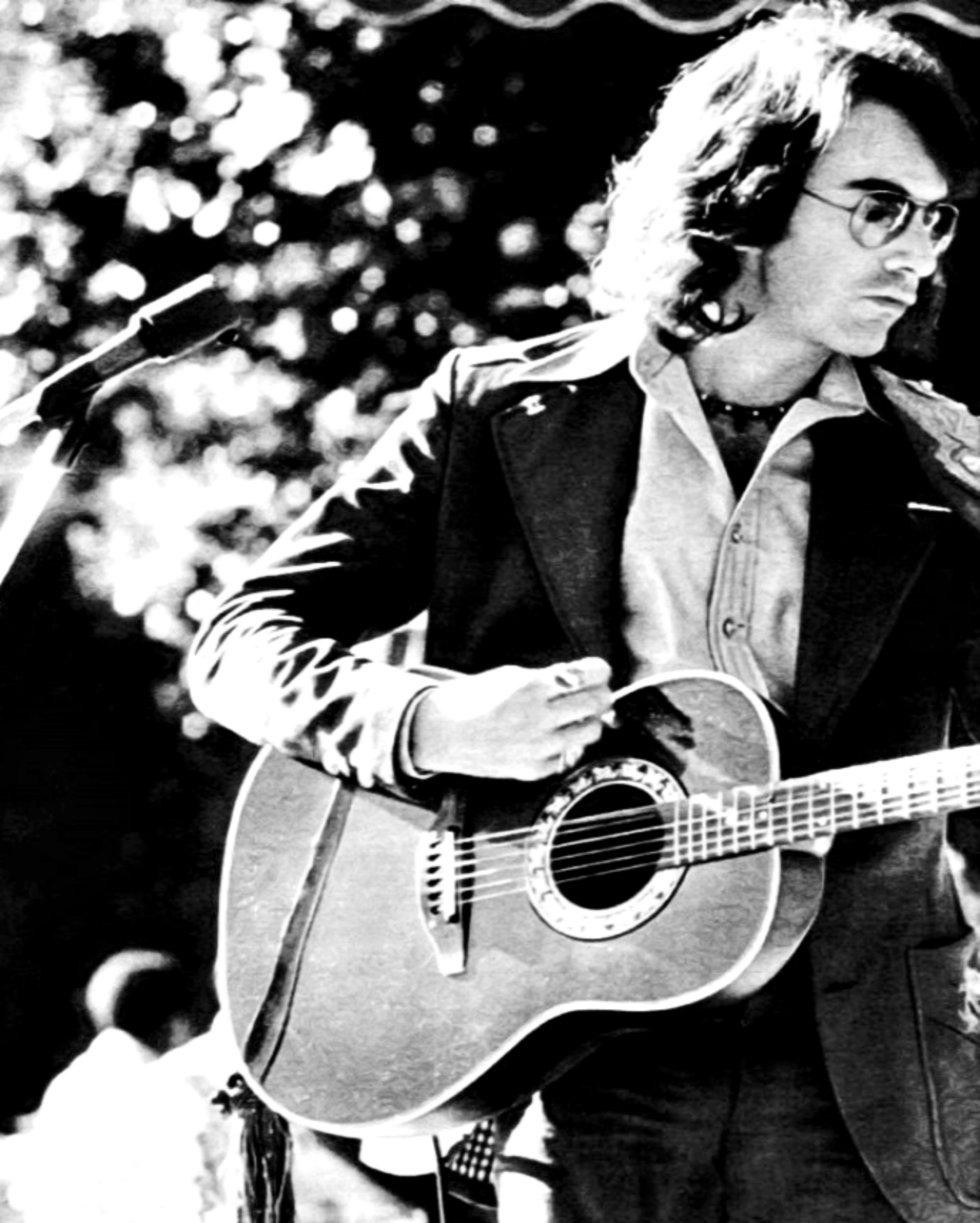This grainy black and white photograph captures a man with long, curly hair, parted at the side, giving off a 70s vibe. He is wearing wide-rimmed glasses and a mustache, and he stands in a casual suit jacket over a collared shirt, which is unbuttoned with a t-shirt underneath. He is in the midst of playing a dark wood acoustic guitar, his fingers adorned with rings, looking poised to strum down. A microphone on a stand is positioned to his left. The scene appears to be outdoors with a hazy background featuring indistinct trees and possibly a faint figure. The lighting is intense, particularly accentuating his shoulder, arm, and hair.